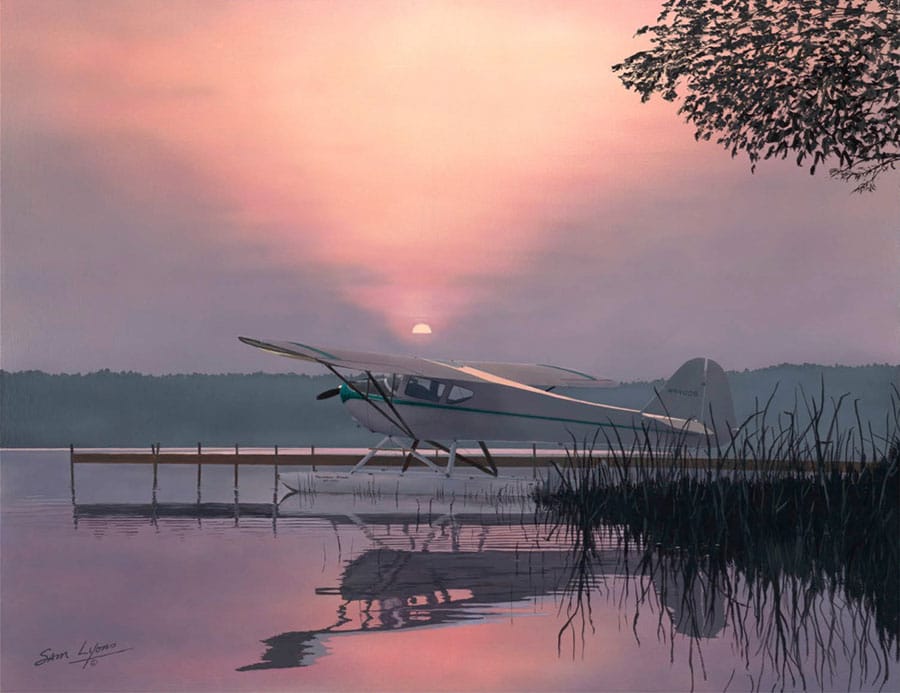This photograph captures the serene moment of a vintage white airplane with a green stripe taking off over a tranquil lake. The scene is bathed in the soft, hazy light of what appears to be sunset, casting a pinkish glow across the sky. The sky, characterized by its reddish pink hue and a striking V-shaped cloud formation, reflects beautifully on the water's surface. In the foreground, tall plants and water lilies emerge from the lake, adding to the natural setting. A long port, resembling a walkway or pier, extends over the water, guiding the viewer's gaze toward the distant hills and mountains that frame the horizon. The entire image exudes a sense of calm, encapsulated by the plane's gentle ascent and its mirrored reflection on the water below.